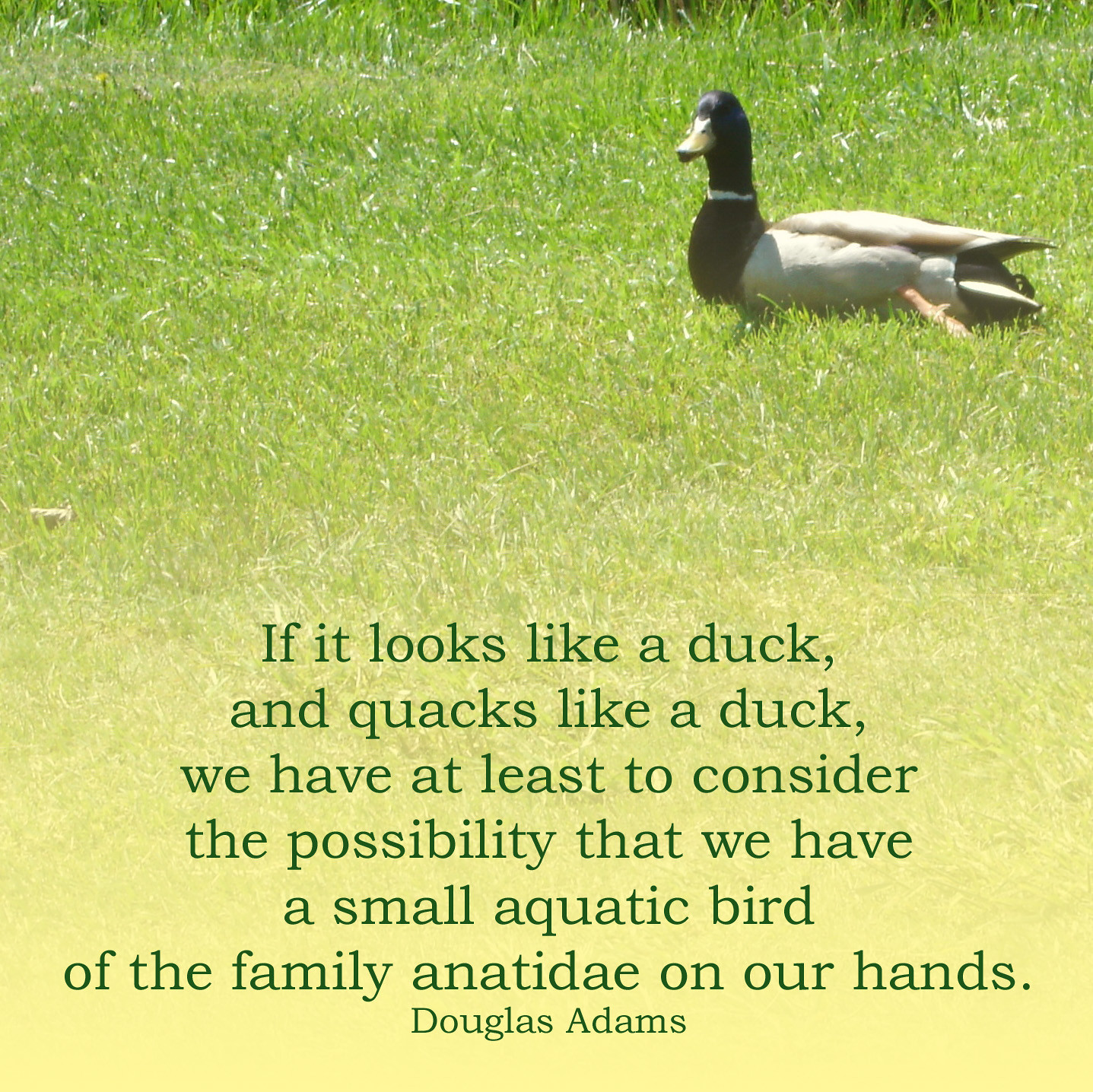The image depicts a duck lying in a grassy field, positioned in the upper right corner facing left with its head turned to the right. The duck has a striking green head, a yellow beak, and a defining white ring around its neck. Its body features a mix of black, brown, and white feathers, with its legs tucked underneath. The grass varies in color, with a yellowish tint at the bottom, gradually turning greener and longer towards the top. At the bottom, in green text that matches the hue of the grass, there is a quote attributed to Douglas Adams: "If it looks like a duck and quacks like a duck, we have at least to consider the possibility that we have a small aquatic bird of the family Anatidae on our hands." The image is set on a sunny day, emphasizing the shine and texture of the grass, and focuses on showcasing the detailed appearance of the duck.